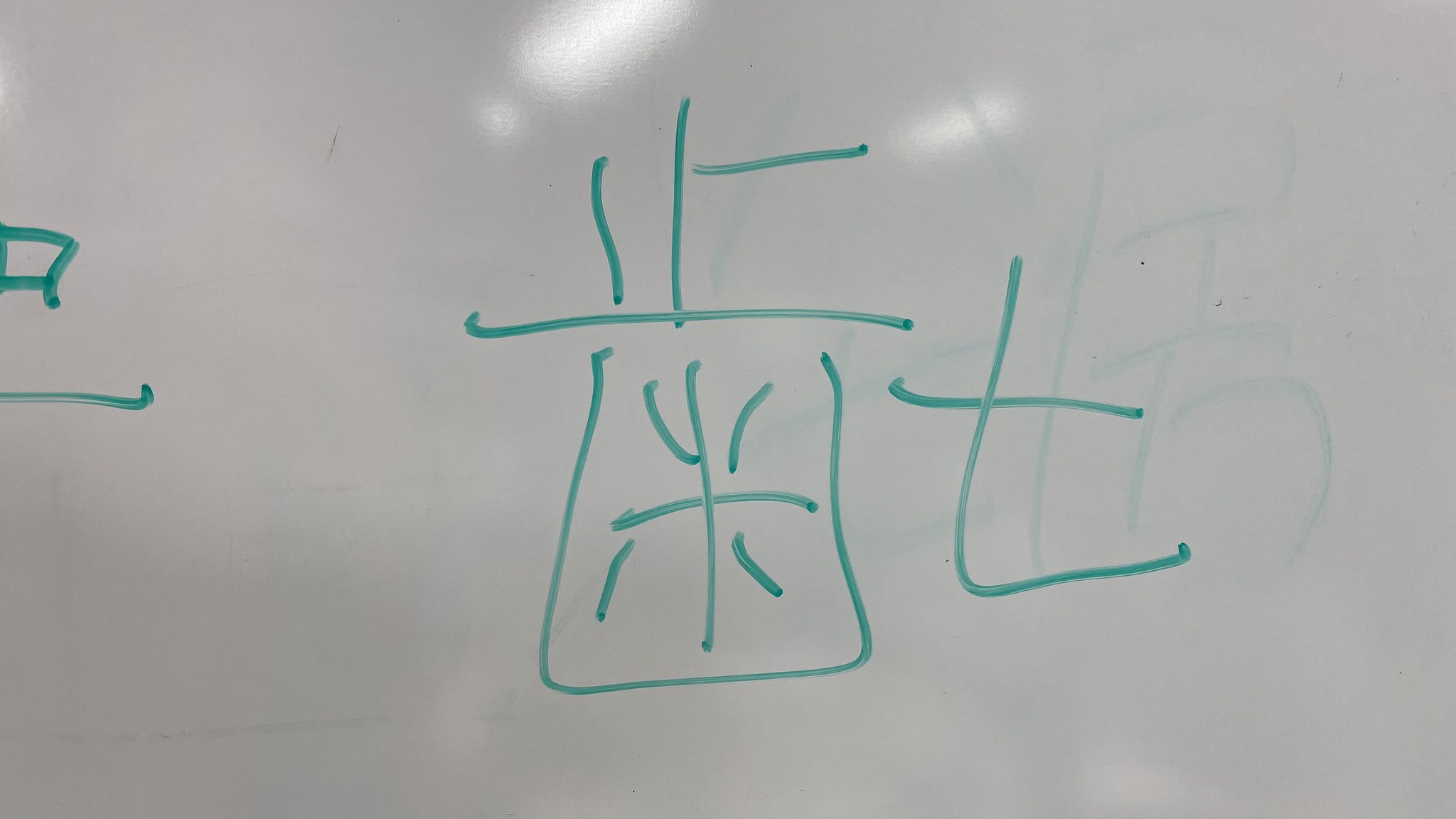This horizontal close-up photograph features a portion of a whiteboard adorned with Oriental symbols etched in green marker ink. The symbols are predominantly centered within the frame, allowing for a detailed examination of their intricate design. To the left of the center, partial impressions of additional symbols peek into view, hinting at a larger composition beyond the image's immediate focus.

The first symbol resembles an abstract depiction of a face topped with a hat, characterized by lines that extend upwards and outwards from the main form. Below this central figure, the shape transitions into the semblance of a plus sign, with diagonal lines converging towards the center, forming a complex, almost face-like structure. The second symbol, simpler in comparison, bears a striking resemblance to a lowercase 't', maintaining a minimalist yet distinct appearance.

These meticulously drawn symbols stand out against the whiteboard's smooth, erasable surface, showcasing the artist's precise control over the green marker. The photograph not only captures the written characters with clarity but also highlights the texture and sheen of the whiteboard, emphasizing its reusable nature.